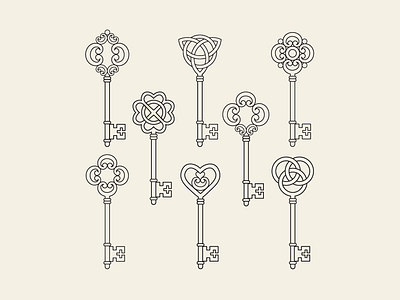This black and white line drawing on an ivory background depicts a collection of eight ornate, old-fashioned skeleton keys. Each key is unique in its intricate top design, showcasing a variety of symbols and interlocking patterns, including a trinity knot, a four-leaf clover, and a heart with an upside-down or tilted C embedded within it. One key features three interlocked circles, while another displays a heart-shaped top. All the keys point to the right, their detailed, lace-like metal craftsmanship evoking a sense of antiquity and Celtic artistry. This detailed illustration, reminiscent of a coloring page, invites viewers to add their own colors to the intricate designs.